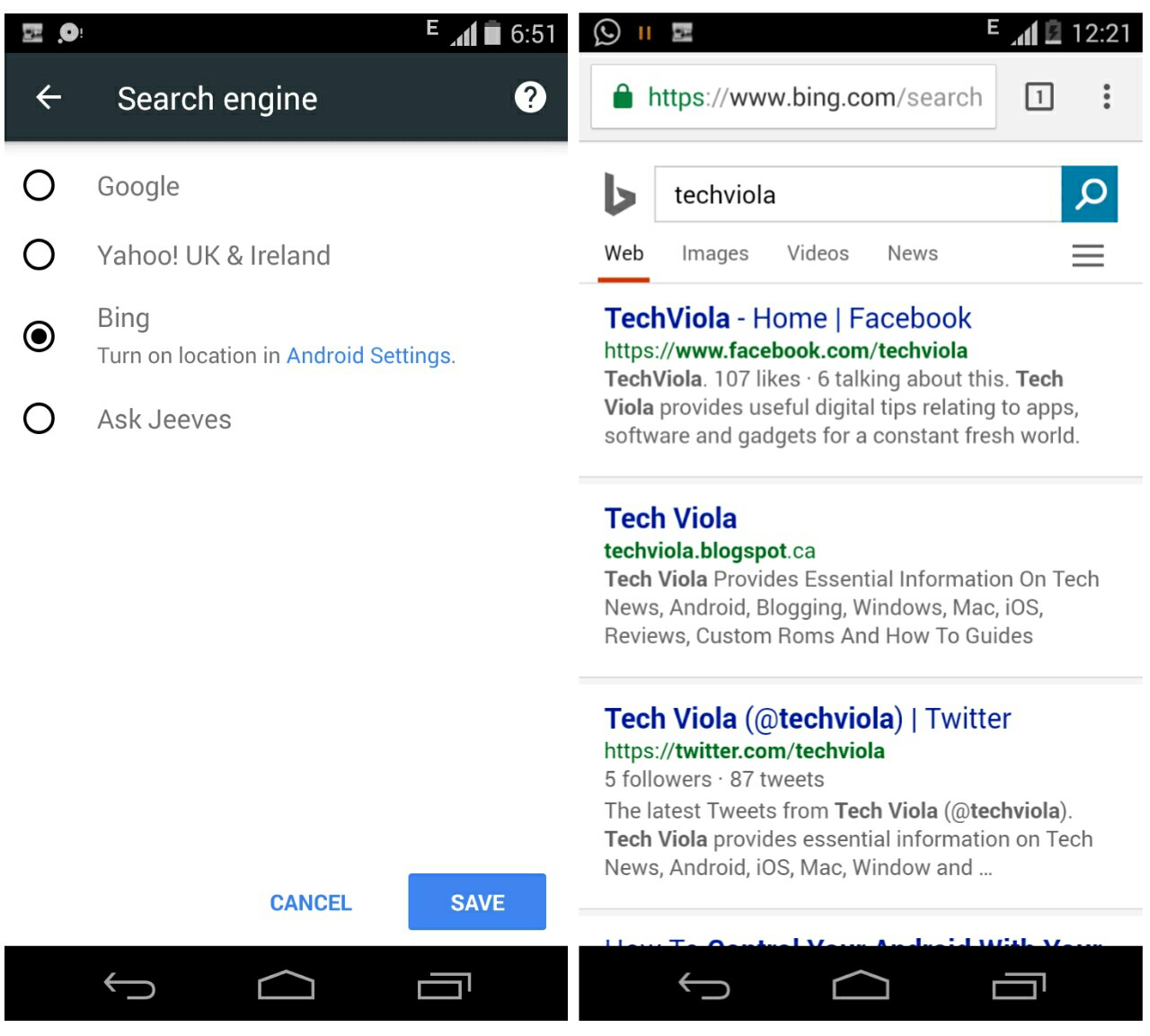This image is divided into two portrait-oriented segments, each resembling a screenshot from a cell phone. Both sections are outlined with a thin white barrier, blending seamlessly into a white background, creating a nearly square overall image.

On the left side, the screenshot indicates a user selecting their preferred search engine. The top of this section features a thin, dark black status bar with four icons: an ascending series of bars likely showing Wi-Fi strength, a battery icon that is nearly full, an "E" symbol for cellular network strength, and the time displayed as 6:51. Beneath this bar, a slightly lighter charcoal grey header holds a left-pointing white arrow next to the text "Search engine" and a white circle with a grey question mark on the far right. Below this, four vertically aligned radio buttons display the options "Google," "Yahoo UK and Ireland," "Bing," and "Ask Jeeves." The third button, next to "Bing," is selected, with an additional notice to "turn on node location in Android settings." At the bottom of the screen, options for "Cancel" and "Save" are available, with "Save" highlighted in a blue box with white text. Another dark black footer below this includes three white icons: a return arrow, an envelope, and two stacked rectangles.

The right side of the image displays a slightly different scene. The top status bar is almost identical to the left image, except the time shown is 12:21, and the battery icon is nearly empty. Instead of a search engine selection interface, this section shows a browser search. The header has a grey background with a white search bar containing a green lock symbol followed by "https://www.bing.com/search." Below, another search bar shows the user has entered "Tech Viola." The Bing logo sits at the left end of this search bar. Beneath the search input, four tabs labeled "Web," "Images," "Videos," and "News" appear, with "Web" highlighted with a red underline.

This section lists three search results:
1. **Top Result**:
   - **Title**: Tech Viola - Home (Facebook)
   - **URL**: https://www.facebook.com/TechViola (in green text)
   - **Description**: Tech Viola 107 likes... (extends over three lines)

2. **Second Result**:
   - **Title**: Tech Viola (BlogSpot)
   - **URL**: techviola.blogspot.ca (in green text)
   - **Description**: Tech Viola provides essential information on tech... (extending over three lines)

3. **Third Result**:
   - **Title**: Tech Viola (@TechViola) - Twitter
   - **URL**: https://twitter.com/TechViola (in green text)
   - **Description**: 5 followers, 87 tweets... (extends over three lines)

This detailed juxtaposition provides a clear depiction of two phone screens in active use, highlighting various elements from a user’s setup preferences to a practical search scenario.